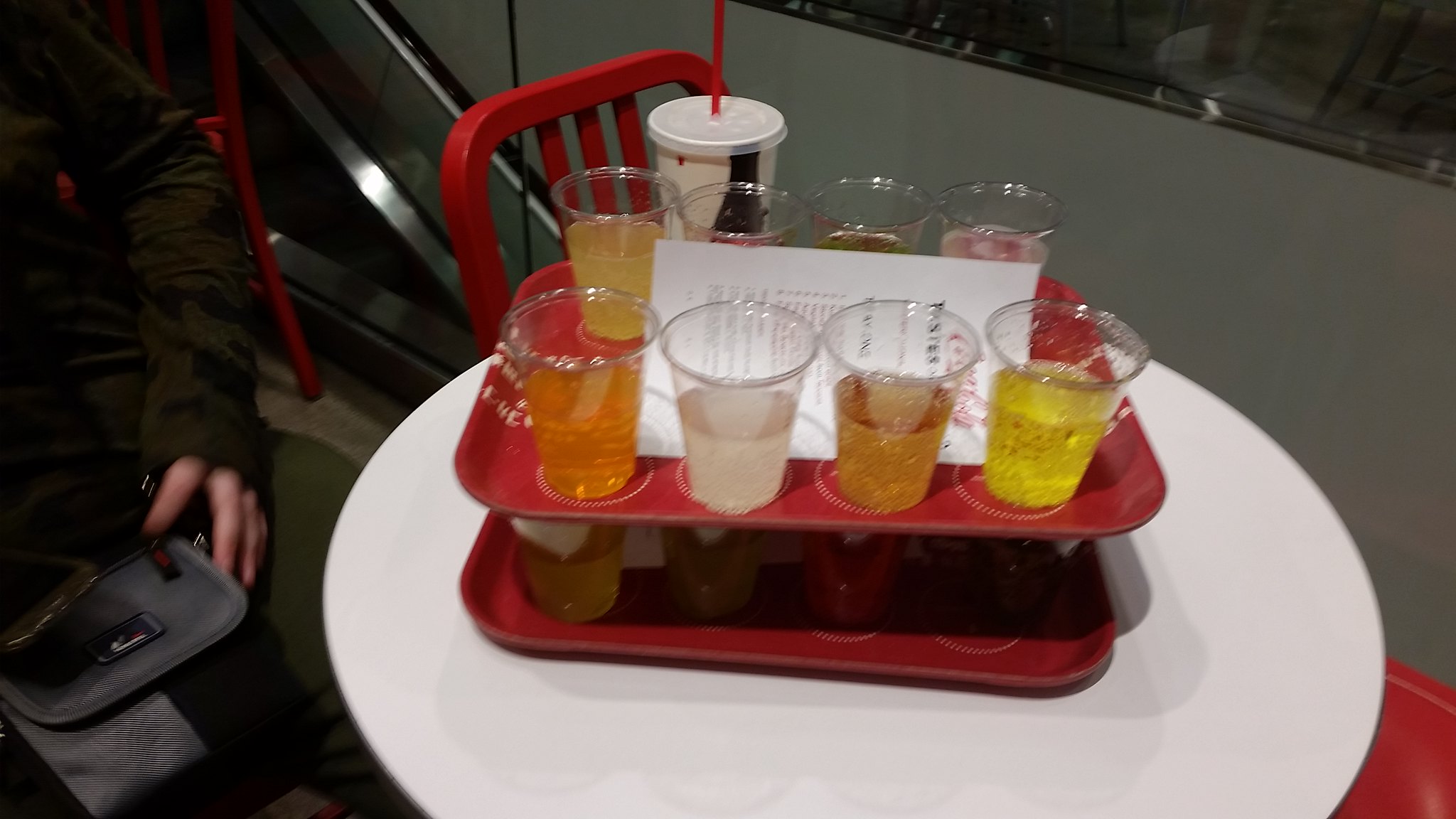In this photograph taken at a restaurant, a scene captures a small white coffee table with a round top, surrounded by red metal chairs. In the background, there is an escalator descending and a gray object, possibly a trash can. The focal point of the image is the table, which holds two red serving trays stacked on top of each other. Each tray contains several plastic cups filled with a variety of differently colored drinks, with hues including bright yellow, amber, white, and orange, suggesting a possible Coca-Cola tasting event. The bottom tray has some cups partially visible, while the top tray is fully balanced on the cups below. Additionally, there is a plastic to-go cup with a red straw positioned towards the back of the table. To the left of the frame, an individual is partially visible, wearing a navy green long-sleeve sweater and matching tights, holding a container and a black folded purse.